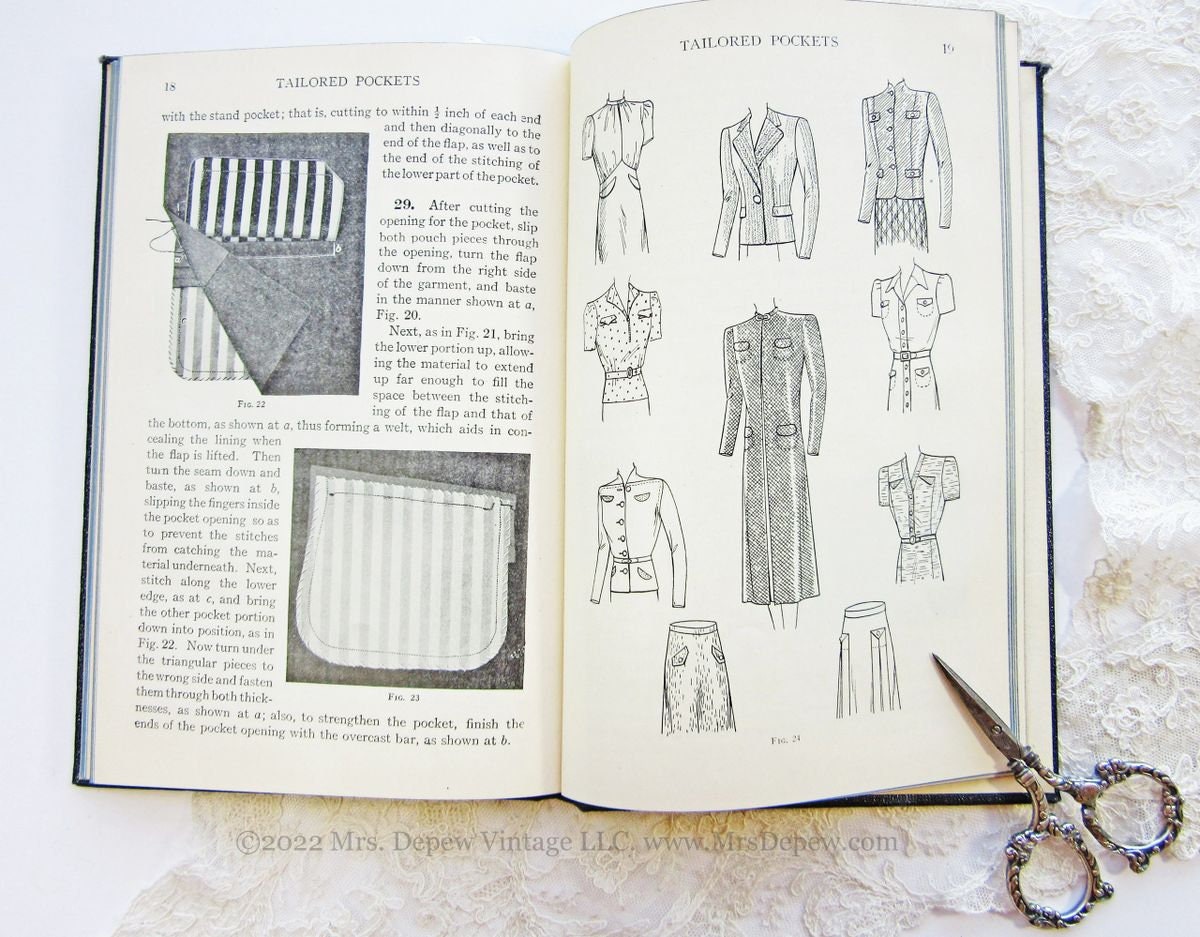This is an image of an open sewing book displaying pages 18 and 19, focused on "TAILORED POCKETS" as indicated by the capital letters at the top of both pages. Resting in the bottom right corner is a dainty pair of ornate, silver sewing scissors with detailed floral or ribbon-like decorations on the handles. Page 18, on the left, is filled with step-by-step instructions and two detailed diagrams, labeled Figures 22 and 23, showing how to construct standard tailored pockets. Page 19, on the right, features illustrations of ten different garments—including jackets, dresses, skirts, a blouse, a suit jacket, a vest, and a trench coat—each showcasing tailored pockets. The bottom of the image includes a watermark that reads "copyright 2022 Mrs. Depew Vintage LLC www.mrsdepew.com."